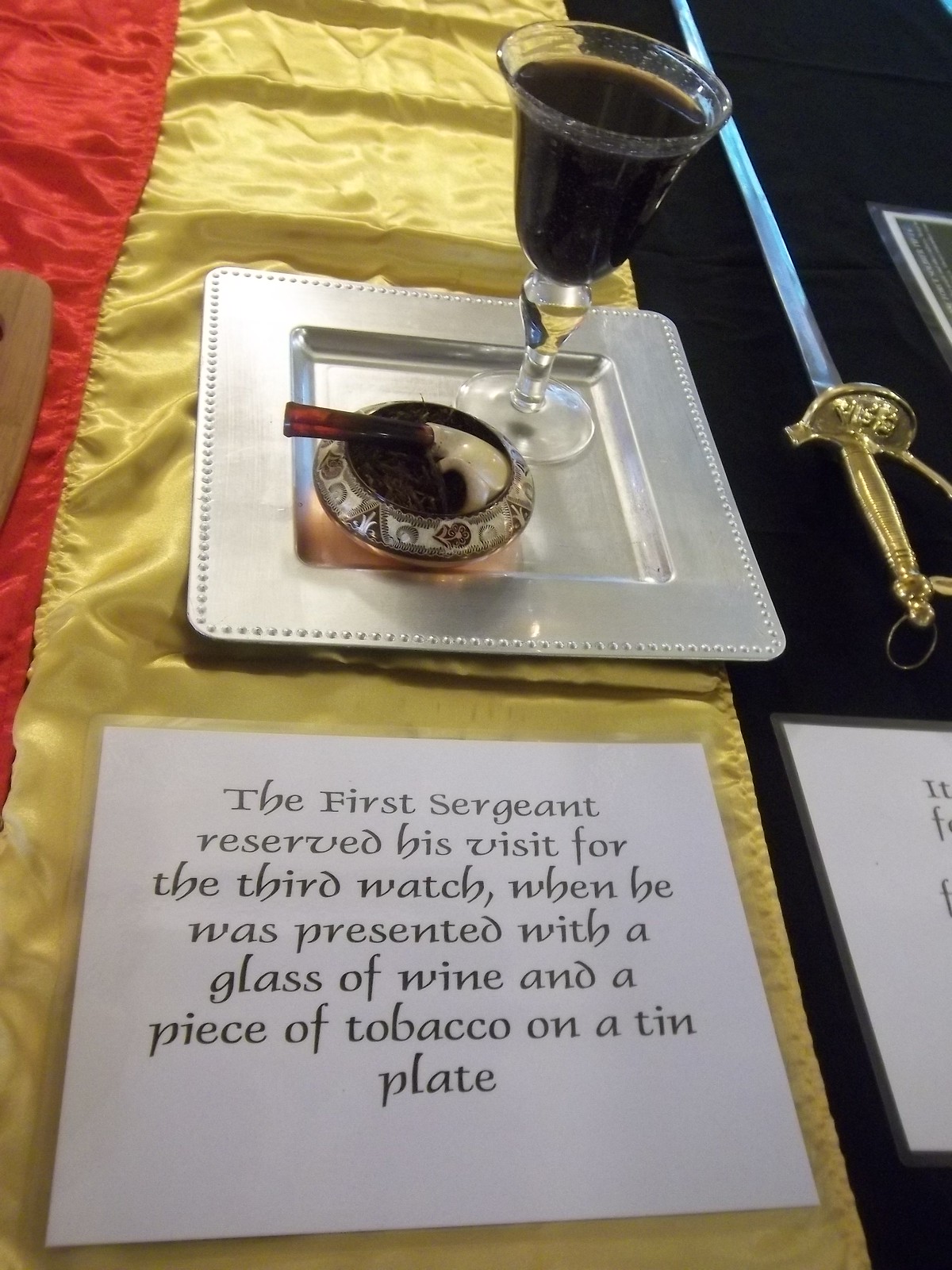The photograph captures a museum exhibit table adorned with luxurious silk materials in red, gold, and dark blue, showcasing an array of historical artifacts. Dominating the upper half of the image is a tin plate displaying a piece of tobacco within a highly decorated pot, alongside a clear glass of wine. The pot, notable for its ornate design, also holds a pipe. Below these items, the artifacts rest on a golden sheet. A prominent laminated sign on white paper provides historical context: "The First Sergeant reserved his visit for the third watch when he was presented with a glass of wine and a piece of tobacco on a tin plate." To the right of the tin plate, a partially visible sword lies on a dark blue section of the silk, featuring a silver blade and a gold handle. Another laminated piece of paper below the sword contains partially readable text. The entire assortment is carefully arranged on what appears to be a black felt table.